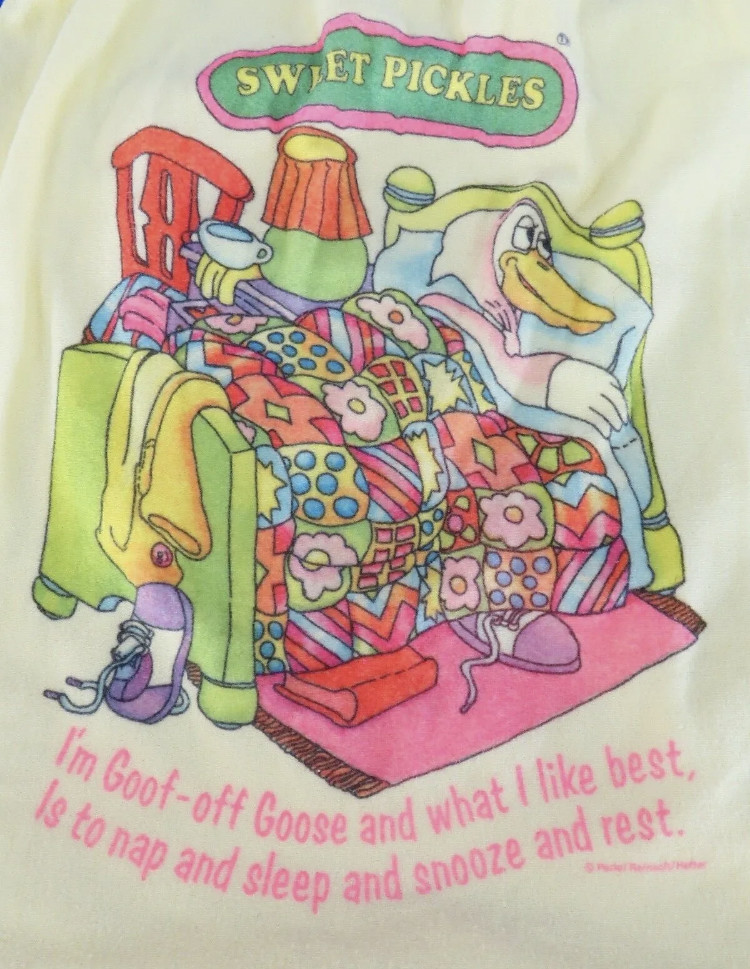This image depicts a whimsical illustration on a t-shirt featuring a grandmotherly white goose with a yellow beak, comfortably nestled in a bed. The goose, dressed in a pink nightgown with a hood, is sleeping on blue pillows and blue sheets. Her quilted comforter is adorned with a vibrant floral pattern in green, pink, yellow, blue, and orange. The bed's headboard and footboard are green with blue accents. Beside the bed, there is a green lamp with an orange shade, a red chair on the left, a purple dresser with a coffee mug on it, and a pink rug with purple and white shoes on top. A yellow jacket hangs over the footboard, and a red book is tucked under the bed. The upper part of the image shows the text "Sweet Pickles" in yellow, outlined in green and pink, while below the goose, it reads, "I’m goof off goose and what I like best is to nap and sleep and snooze and rest." This colorful and detailed scene seems to be part of a children's clothing design.